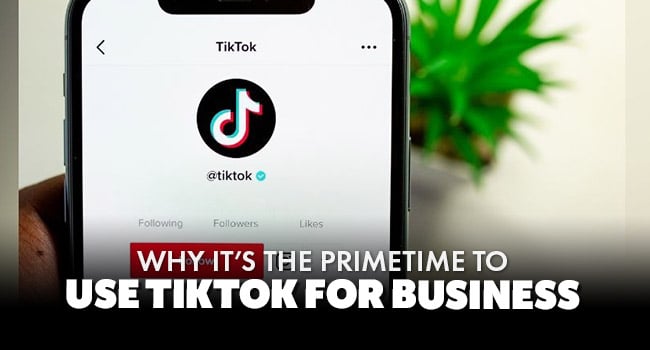This image captures a TikTok advertisement prominently displayed on a smartphone screen. The phone screen shows the TikTok app, identifiable by its iconic musical note logo with a curved edge, which is also verified. The interface displays various segments including 'Following,' 'Followers,' and 'Likes.' 

In the background of the image, there is a lush green plant set against a beige or whitish wall, adding a touch of freshness to the scene. The backdrop also includes a wood grain table or surface, providing a natural and organic element to the composition.

Overlaying the picture, at the bottom, there is a salient text in all capital letters that states: "WHY IT'S THE PRIME TIME TO USE TIKTOK FOR BUSINESS." The phrase "WHY IT'S THE PRIME TIME TO" appears in slightly smaller font, while "USE TIKTOK FOR BUSINESS" is emphasized in a thicker, more robust font. Additionally, behind the word "WHY," there is a red rectangle from the TikTok page interface, drawing attention and adding a pop of color.

Subtle shadows cast by the plant and the other objects in the picture enhance the depth and realism of the scene.